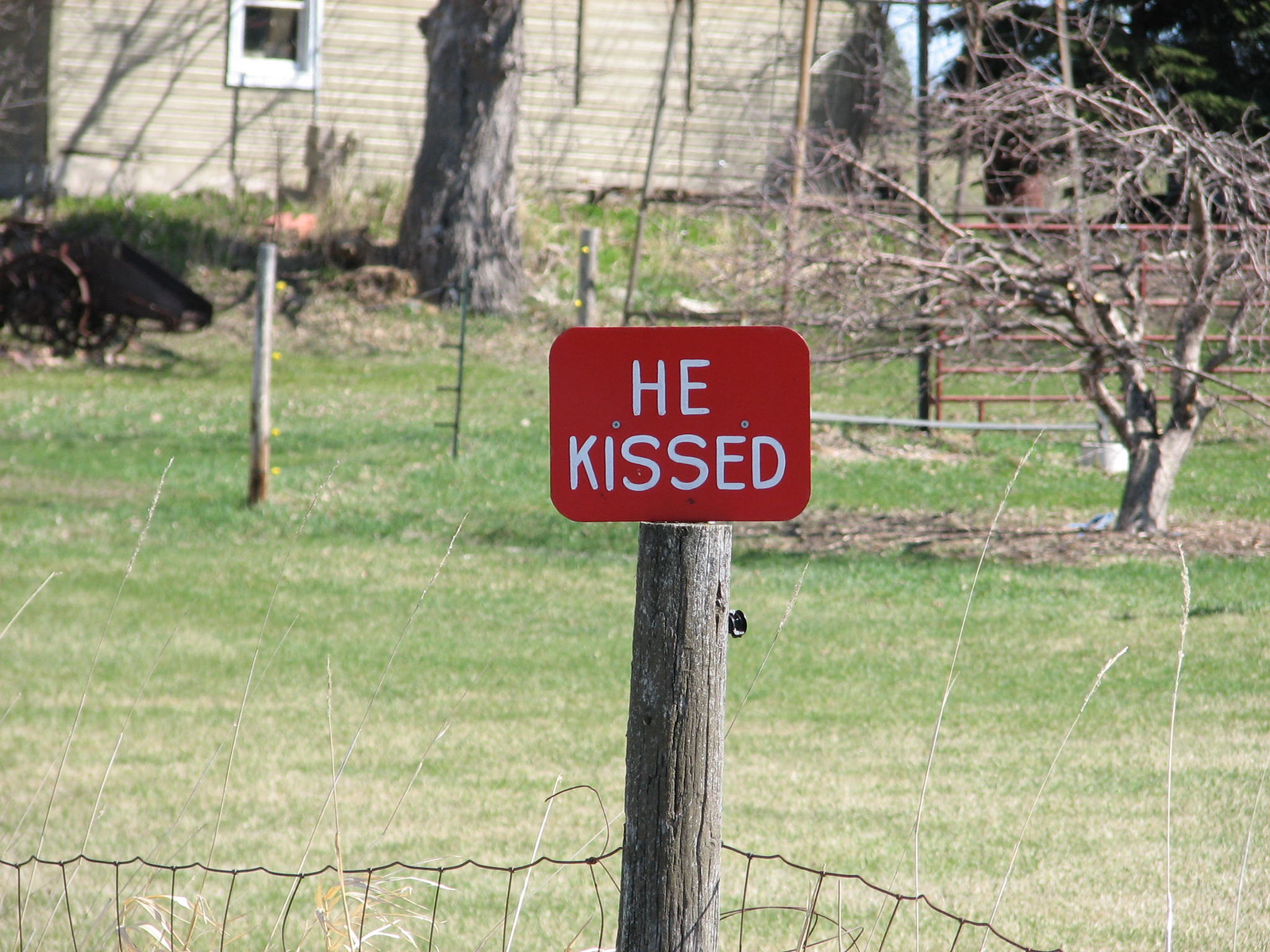In this image, a weathered wooden post serves as a support for a wire fence. Midway up the post, it becomes a bare, brown wood fixture, ascending to a small, red rectangular sign with its shorter side vertically aligned. The sign features white letters that read, "He Kissed." Surrounding the post is a vibrant scene of green grass interspersed with patches of yellow grass and scattered yellow dandelion flowers. In the backdrop, a small, leafless light-brown tree with wide branches adds a stark contrast against the foliage. Further back stands a beige-colored house adorned with white window trim and a visible window. Additional visual elements include another brown tree and a metal pole, with its lower portion rusted, transitioning to a silver or gray color at the top.